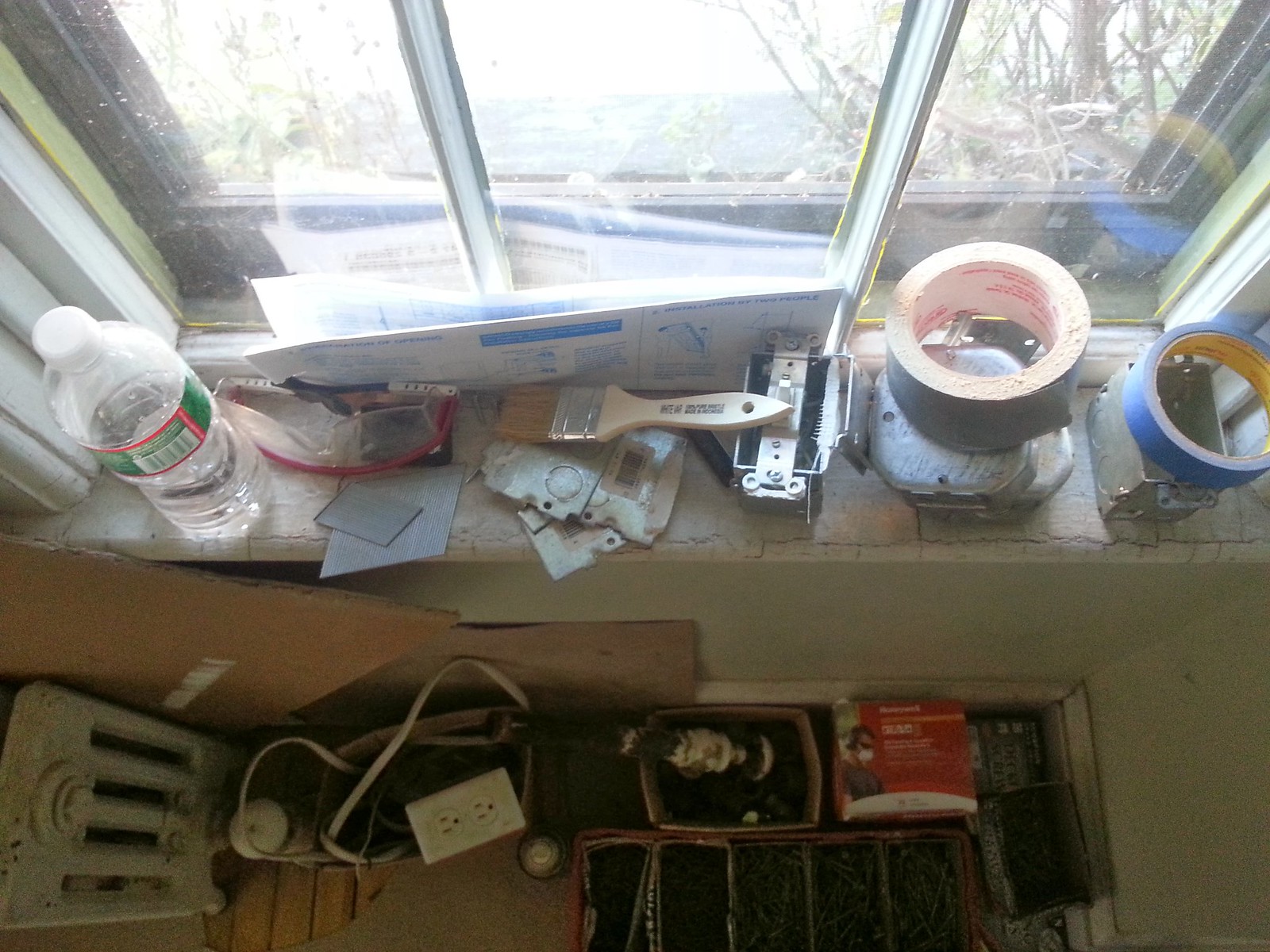An aerial view of a well-worn windowsill, cluttered with various tools and objects, each telling a story of recent work. On the left side of the windowsill lies a half-full water bottle adorned with a green label, keeping a gray roll of duct tape company. Moving to the right, a beige paintbrush with brown bristles rests casually in the middle of the frame, flanked by a roll of blue tape sitting to the far right. Below the dusty, crack-ridden, light-colored windowsill, the floor hosts a light power outlet and several boxes filled to the brim with screws or nails. Through the upper panes of the window, daylight streams in, casting a natural glow over the scene while branches from nearby trees subtly frame the window, hinting at the world outside. A piece of cardboard nestles against the bottom of the wall, further adding to the sense of a space in the midst of activity and transformation.